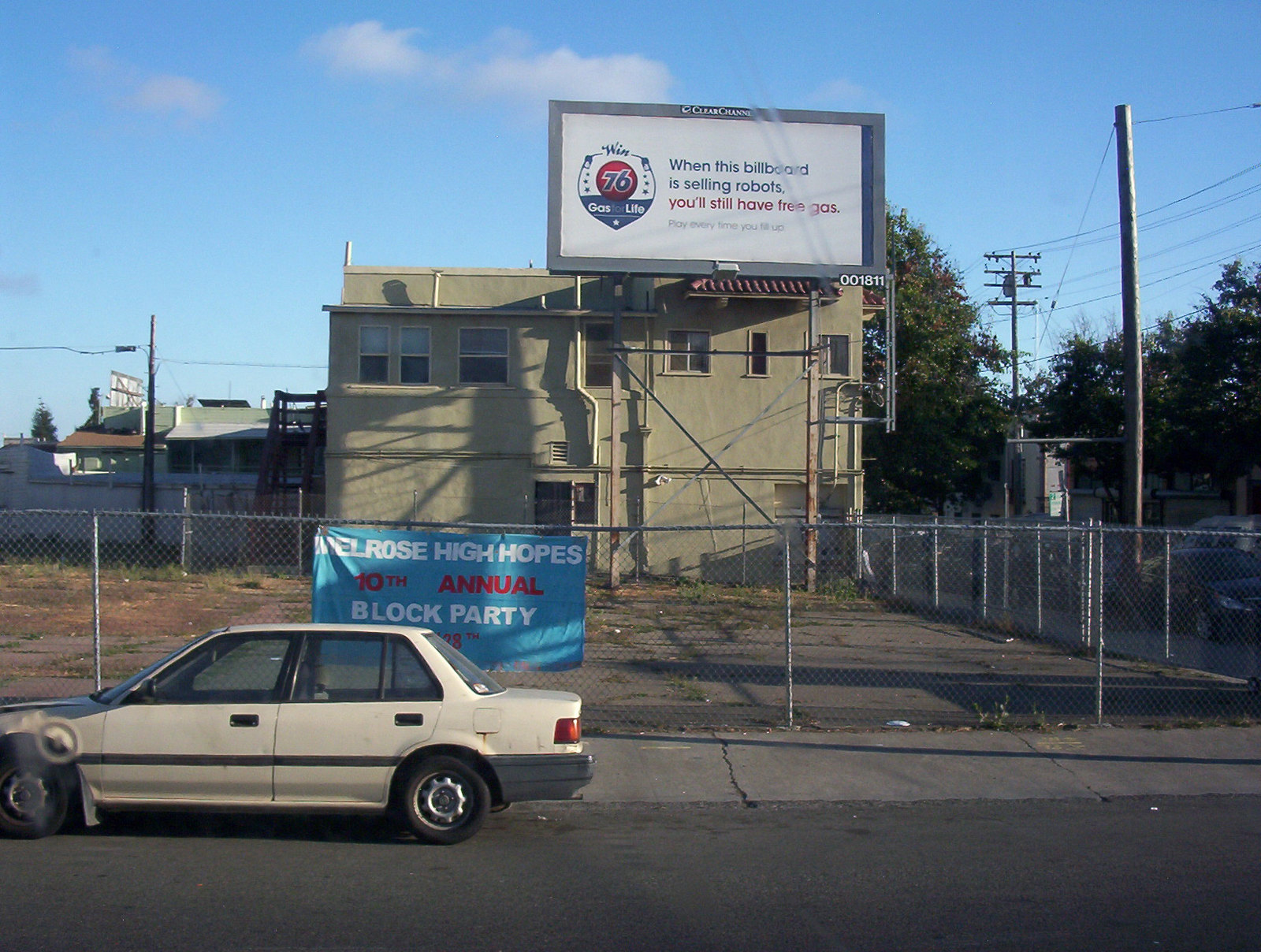The photograph depicts a city street scene with a prominent billboard atop a building. The billboard reads, "When this billboard is selling robots, you'll still have free gas. Win number 76 Gas Life." Below the billboard, there is a vacant lot featuring patches of dirt, weeds, and some areas of paved asphalt. This lot is enclosed by a chain-link fence, adorned with a baby blue banner. The banner, with white and red lettering, announces the "Melrose High Hopes 10th Annual Block Party." However, part of the banner's text is obscured by a cream-colored, 1990s-era Honda, which is parked in front of it. The car appears to be in poor condition and is unoccupied. Surrounding the scene are electricity poles, streetlights, and several trees, indicating that the area might be residential or multi-use.